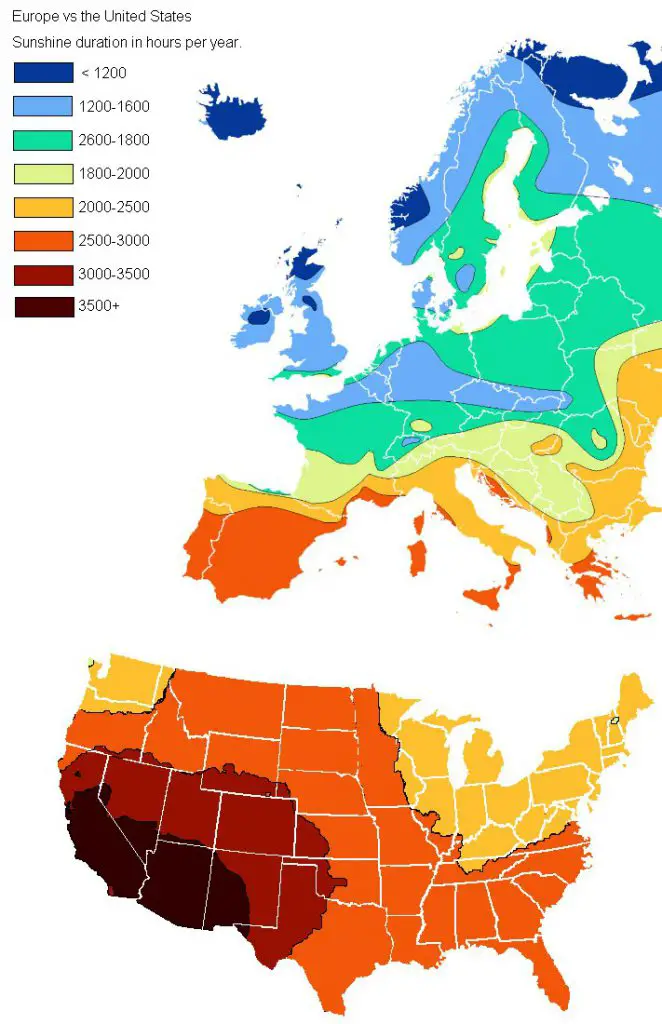The image depicts a detailed heat map titled "Europe versus the United States: Sunshine Duration in Hours per Year" in black text at the upper left corner. This comparative map charts annual sunshine durations for the United States and Europe, with the U.S. map positioned on the bottom and Europe's on the top. An accompanying color guide on the left side of the image correlates multiple colors to specific ranges of sunshine hours. For instance, dark blues indicate regions with less than 1200 hours of sunshine, while dark browns and reds represent areas with over 3500 hours. 

In the United States, regions like California, Arizona, New Mexico, and parts of Nevada and Utah are depicted in dark reddish-browns, indicating they receive upwards of 3500 hours of sunshine per year. The color gradient shifts through lighter reds, oranges, and yellows as it moves eastward, showing a decrease to around 2000-2500 hours on the East Coast. Conversely, the European map shows a predominance of dark and light blues in countries like France, Germany, and England, signifying 1000-2000 hours of sunshine annually, with even less sunshine in Scandinavia. However, southern Europe, particularly Spain and Portugal near the Mediterranean, is marked with brighter colors like yellows and lighter oranges, highlighting higher sunshine durations of 2000-3000 hours annually.